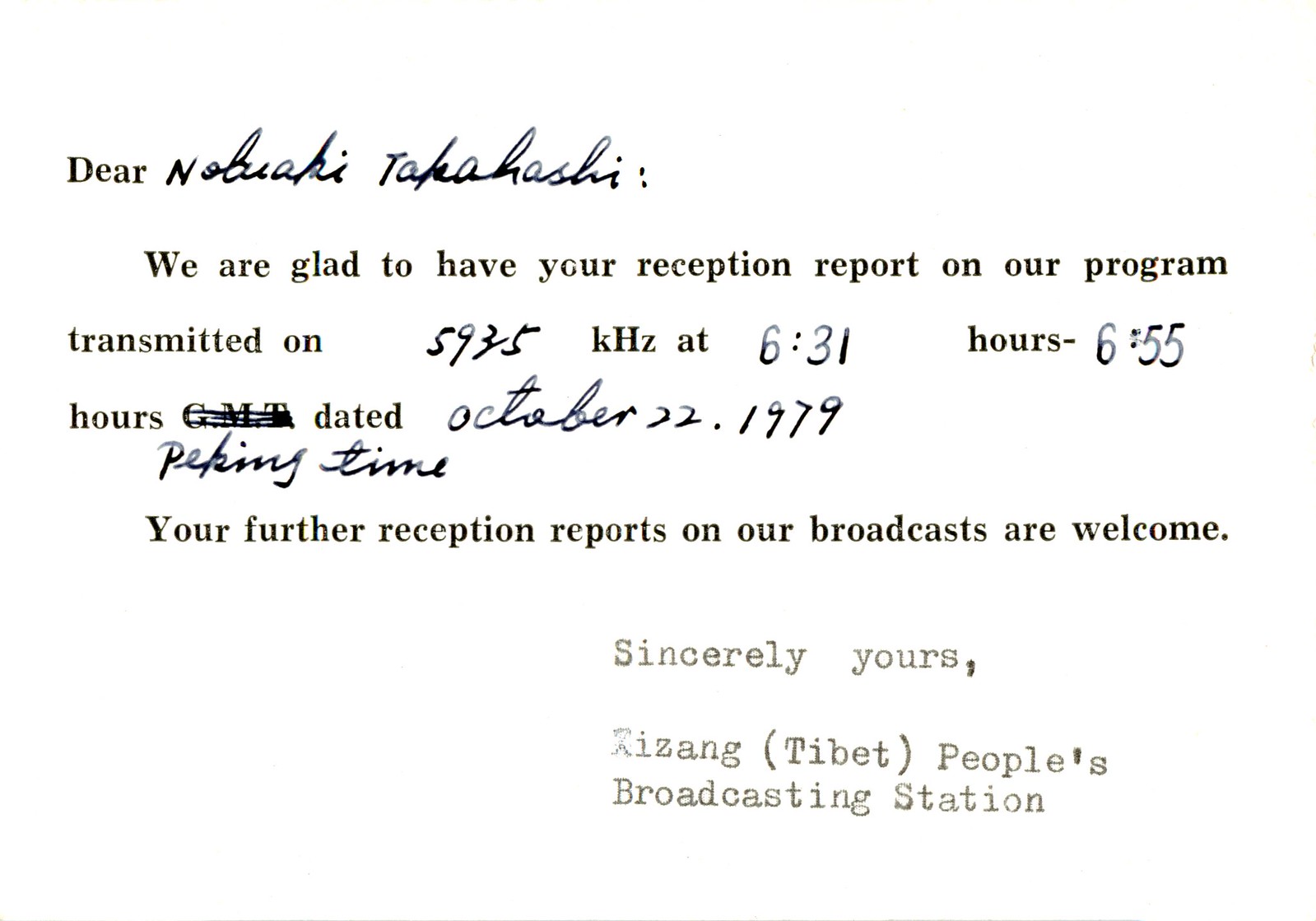This image appears to be a digital scan of a white piece of paper with both printed and handwritten text in black ink. The top left of the document starts with the printed word "Dear" followed by the cursive handwritten name "Nobiyuki Takahashi." The document continues with printed text stating, "We are glad to have your reception report on our program transmitted on." In the next line, the handwritten frequency "5935" is noted next to the printed "KHZ" at "6:31," followed by handwritten "hours" and "6:55" denoting the broadcast times. Below this, the pre-printed "GMT" has been crossed out and replaced with the handwritten note "Peking time." The pre-printed "Dated" is completed with the handwritten date "October 27, 1979." Towards the bottom, the document extends a courteous message, "Your further reception reports on our broadcasts are welcome." Finally, the document is stamped with "Sincerely yours, Xizang (Tibet People's Broadcasting Station)." A thin strip along the bottom and right edge of the image suggests it is a photocopy.